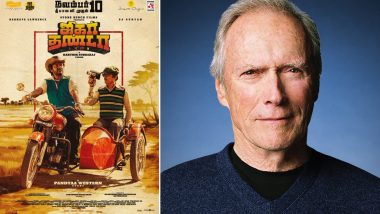The image is a split picture featuring a movie poster on the left and a photograph of Clint Eastwood on the right. The movie poster is designed in a foreign language and depicts a man in a cowboy hat, green vest, and white undershirt riding a red motorcycle with a sidecar. The sidecar is occupied by another man wearing a striped vest and a beret, who appears to be videotaping with a camera. The overall background of the poster has a yellowish tone with grass and trees visible. The photograph on the right shows Clint Eastwood, likely aged around 65 to 70, wearing a blue sweater with a black undershirt, set against a blue background. This combined scene suggests a nostalgic reference to a film, albeit the specific details remain unclear due to the non-English text.